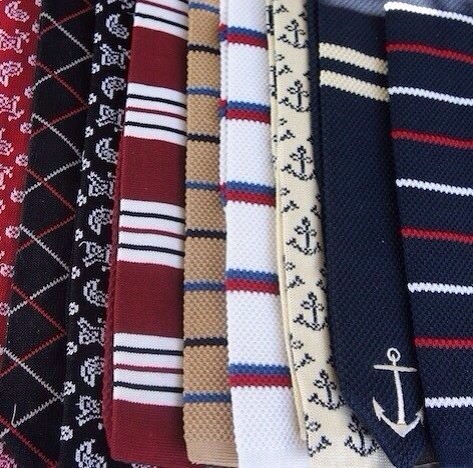This photograph showcases an array of various fabrics, each thoughtfully layered on top of the other in a cohesive manner, suggesting they might be part of a collection. The fabrics share a narrow, rectangular shape common to neckties, though they could also be towels or placemats. The color palette includes vibrant reds, blacks, blues, whites, and beiges, each adorned with unique patterns such as paisleys, crisscross designs, and stripes, as well as charming motifs like anchors. From left to right, the fabric designs include:

1. Red with white symbols.
2. Black with red and white diamond patterns.
3. Black with distinctive white patterns.
4. Red with a blend of white, blue, and red stripes.
5. Tan with both dark and light blue stripes.
6. White with dark blue and red stripes.
7. Tan with black anchor motifs.
8. Blue with tan stripes and a white anchor.
9. Navy blue with red and white stripes.

The close-up perspective of the image intricately captures the detailed designs and textures of each fabric piece, highlighting the rich variety and the harmonious blend of colors and patterns.